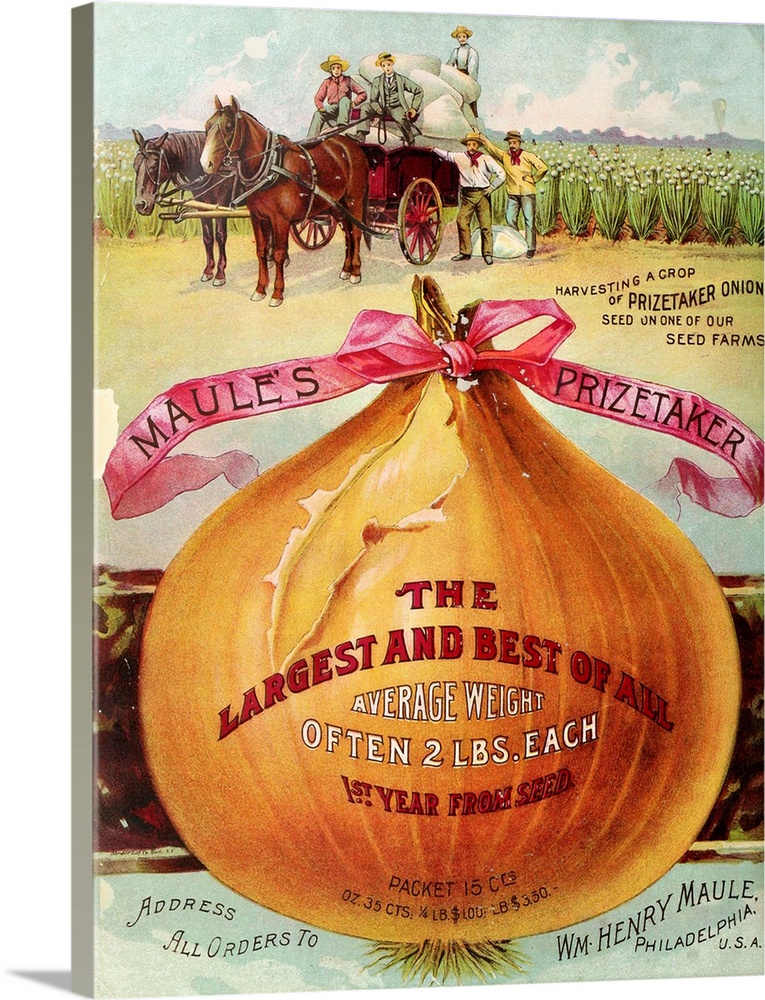This vintage advertisement, likely from a 1910s to 1930s magazine, is illustrated on a canvas or board. The ad features a vivid and detailed scene centered around a colossal onion adorned with a red ribbon labeled "Mall's Prize Taker." Text on the onion boasts, "The largest and best of all, average weight often two pounds each, first year from seed, packet 15 cents, ounce 35 cents, quarter pound $1.00, pound $3.50."

Above the onion, a lively farm scene unfolds under a clear blue sky. Two horses, one brown and one red, pull a wagon laden with sacks of onions. Five men, dressed in attire reminiscent of the 1880s, are depicted: two at the reins, one standing atop the wagon bed, and two on the ground, hands resting against the wagon. Behind them, rows of onion plants stretch into the horizon, indicating a bountiful harvest.

At the top of the advertisement, additional text reads, "Harvesting a crop of Prize Taker onion seed on one of our seed farms." At the bottom, more sky is visible along with the address for orders: "W.M. Henry Mall, Philadelphia, USA." The entire composition captures the essence of early 20th-century agricultural pride and marketing flair.